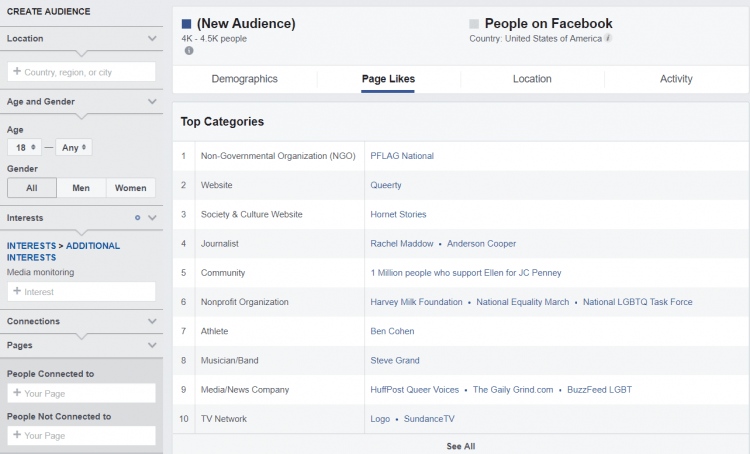The image depicts a 'Create Audience' section of a website with a primary focus on audience targeting. The left-hand side of the page is shaded in gray and features several fields for user input categorized as 'Location' (where you specify your country, region, and city), 'Age and Gender,' 'Interests' (with options for primary and additional interests highlighted in blue), and 'Connections' (detailing pages, people connected to, and people not connected to).

The main content area of the page has a lighter gray background and is titled 'New Audience.' It provides demographic information specifically for 'People on Facebook' located in the 'United States of America,' with an estimated audience size of '4,000 to 4.5 thousand people.'

Further breakdowns of the audience include sections on 'Demographics,' 'Page Likes,' 'Location,' and 'Activity.' The 'Page Likes' section features a bold bar labeled 'Top Categories,' listing various interests ranked from one to ten. These categories include:
1. Non-Governmental Organization
2. Website
3. Society and Cultural Website
4. Journalist
5. Community
6. Nonprofit
7. Athlete
8. Musician Band
9. Media News Company
10. TV Network

Next to each category, there are names or groups written in blue, signifying specific entities or individuals under 'People Likes,' which is the currently active and underlined section, indicating its focus in this instance. There is limited to no information under the other sections.

Overall, the image illustrates the process of targeting a specific audience by filling out detailed criteria to refine and identify your target demographic effectively.